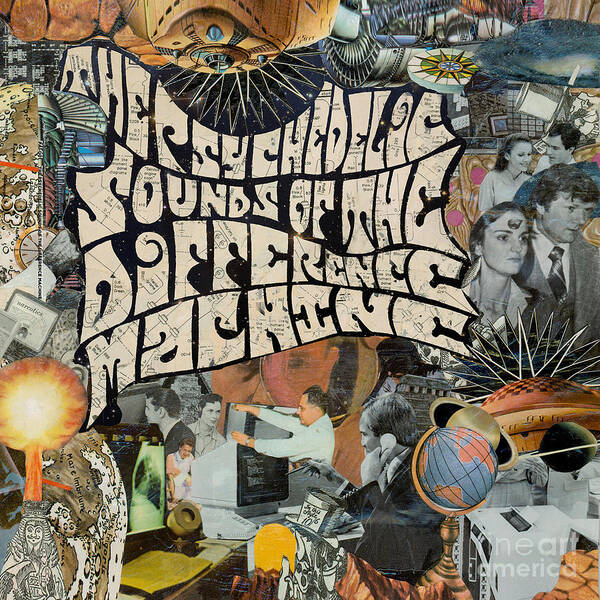The image is a busy, intricate collage that combines both color and black-and-white pictures, creating a visually dense composition. Dominating the center-top of the image are off-white letters spelling out "The Psychedelic Sounds of The Difference Machine." Scattered all over the background are various random pictures that include a globe of the world, a man at a computer with an old-fashioned, boxy monitor, heads and faces of multiple people, both men and women, and a newspaper. In the collage, there's a noticeable presence of people from different time periods; one man in a suit reminiscent of the 1970s with a large tie, and a woman beside him with something on her forehead and a collared shirt. Another prominent image is of a man seemingly fixing a computer, accompanied by a black-and-white photo of a man on a telephone and a couple. The bottom-right corner of the image features faint, light white text that reads "Fine Art America." The collage give an impression of random, overlapping magazine clippings arranged to create a chaotic yet intriguing artwork.